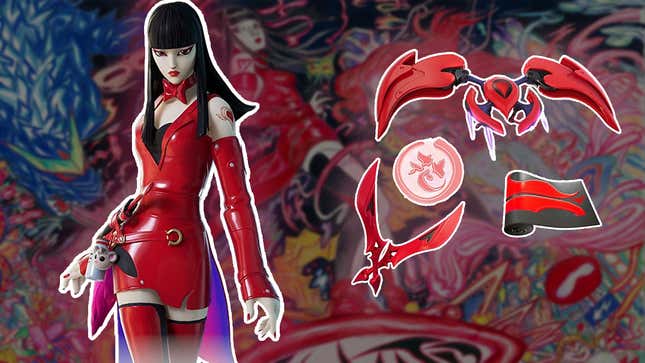The image showcases a detailed vinyl collectible, depicting a stylized anime or manga character of a woman clad in an all-red ensemble. She wears a short red leather dress with matching arm coverings, red leggings, and a red leather bow tie. Her striking appearance is highlighted by her dark hair, red lipstick, and a red heart tattoo on her shoulder. Hanging from her belt is a hip bag adorned with a small container featuring an animal face, perhaps a kitten keychain or charm. To her right, there are several accessories possibly intended for the figurine. These include a head adornment with impractical, large anime-style horns, a red and white token with unrecognizable symbols, a small black and red scroll, and what appears to be a weapon or boomerang resembling her bow tie. Additionally, there are two crossed red daggers and a circular item with red scribblings on it. The background consists of multicolored, blurred artwork depicting an artistic rendition of the same character, enhancing the overall impression of a highly detailed and playful scene, possibly part of a video game avatar or collectible series.